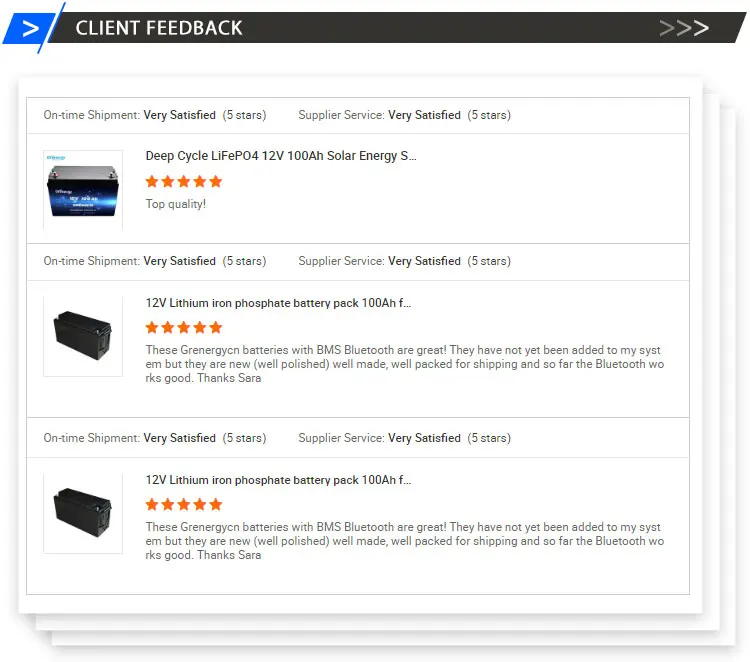In this image, the top left corner features a small blue rectangle with a white arrow pointing to the right, accompanied by the text "client feedback." On the top right, there are three right-pointing arrows: the one on the far right is white, the middle one is gray, and the one on the left is a darker gray. 

At the center of the image, three products are showcased. The top middle product is labeled "DeepCycle Life PO4 12V 100AH Solar Energy" with a five-star rating in orange, followed by the text "top quality." To its left is an image of the product, a black box-shaped item. 

Below this product is another labeled "12V Lithium Iron Phosphate Battery Pack 100AH," also boasting a five-star rating, with a similar black box-shaped image to the left. The final product, positioned at the bottom middle, bears the same label "12V Lithium Iron Phosphate Battery Pack 100AH" along with a five-star rating and identical black box-shaped imagery on its left.